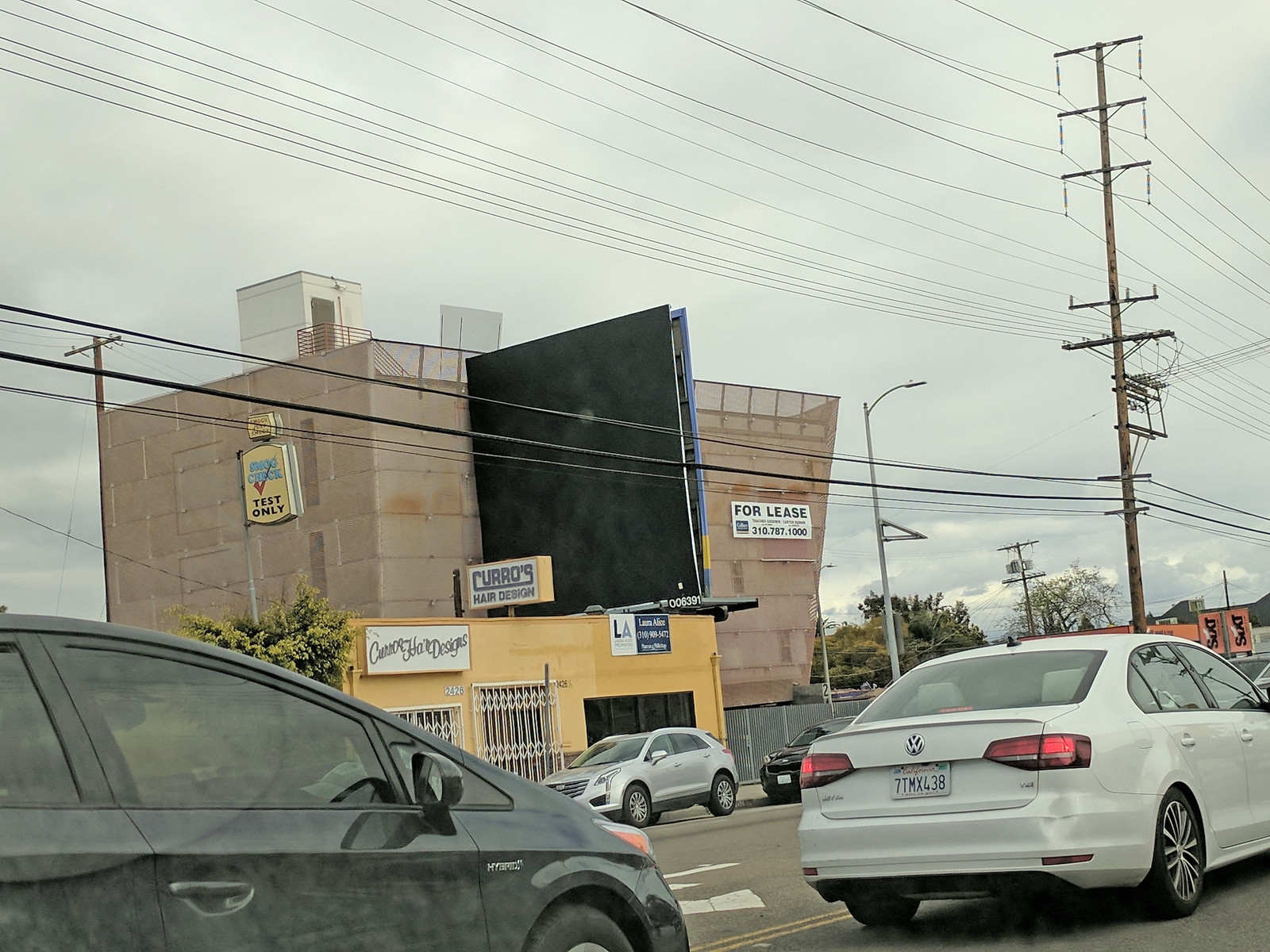In this outdoor daytime photograph taken under a hazy, cloudy sky, we gaze towards the center background where a large tan building stands, spanning three or four stories. The building features a prominent black square projection, likely a defunct sign, and a white rectangular sign to its right that reads "For lease" along with a phone number. In front of this building is a smaller, one-story mustard-yellow structure bearing the name "CURROS Hair Design" on a sign above it; the windows and doors of this establishment are secured with bars. The foreground depicts street traffic, including the right side of a white Prius and the rear end of a dusty black Volkswagen four-door sedan with the license plate 7TMX438. A tall utility pole with numerous utility lines dominates the upper right corner of the image, stretching across the frame from the upper left to the lower right. In the distance, additional cars line the road, providing context to this bustling urban street scene. Scattered trees are also visible, contributing to the city's landscape.